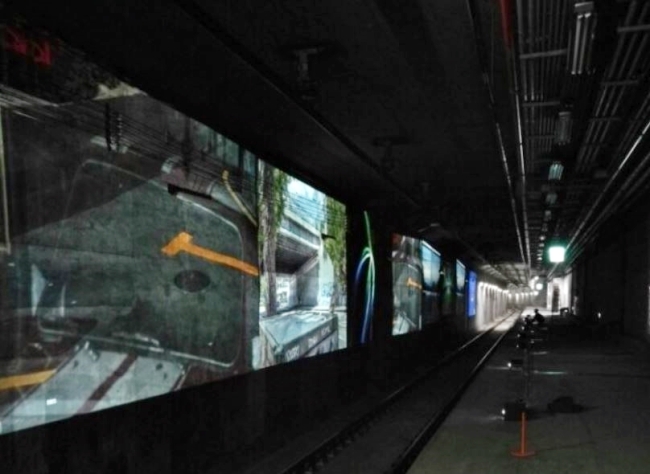The image depicts a dark, underground subway tunnel, likely abandoned, with a single railway track running through it. The ceiling is lined with metal pipes extending into the distance. On the left wall, several projectors display a series of images, including structures, an outdoor setting with trees, and abstract designs resembling a Mac screensaver with green lines and 3D shapes. The projectors create a makeshift art installation. The floor is gray and the overall impression is one of neglect, characterized by the dim, almost pitch-black surroundings. The tunnel interior is punctuated by a distant, brightly lit area further down the path, creating a stark contrast with the immediate gloom.